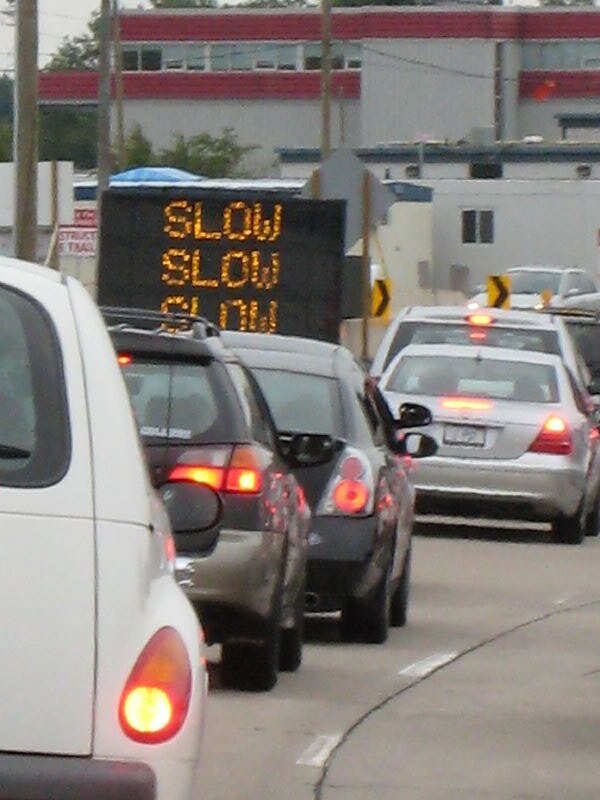This image captures a city street scene from the vantage point of a passenger seated in the back of a car, positioned at the end of a line of vehicles. The right-side view reveals the rear ends of approximately five cars, all with their brake lights illuminated. A prominent black sign with bold yellow letters stating "SLOW, SLOW, SLOW" is situated about midway to the left side of the frame. In the background, several large cement buildings, appearing industrial in nature, dominate the skyline. One notable building features a distinctive design with a red horizontal section at the top, followed by a row of windows, and another red stripe below them. The road directly ahead shows a dotted middle line, further emphasizing the stop-and-go traffic. The overall mood encapsulates a typical scene of urban congestion.